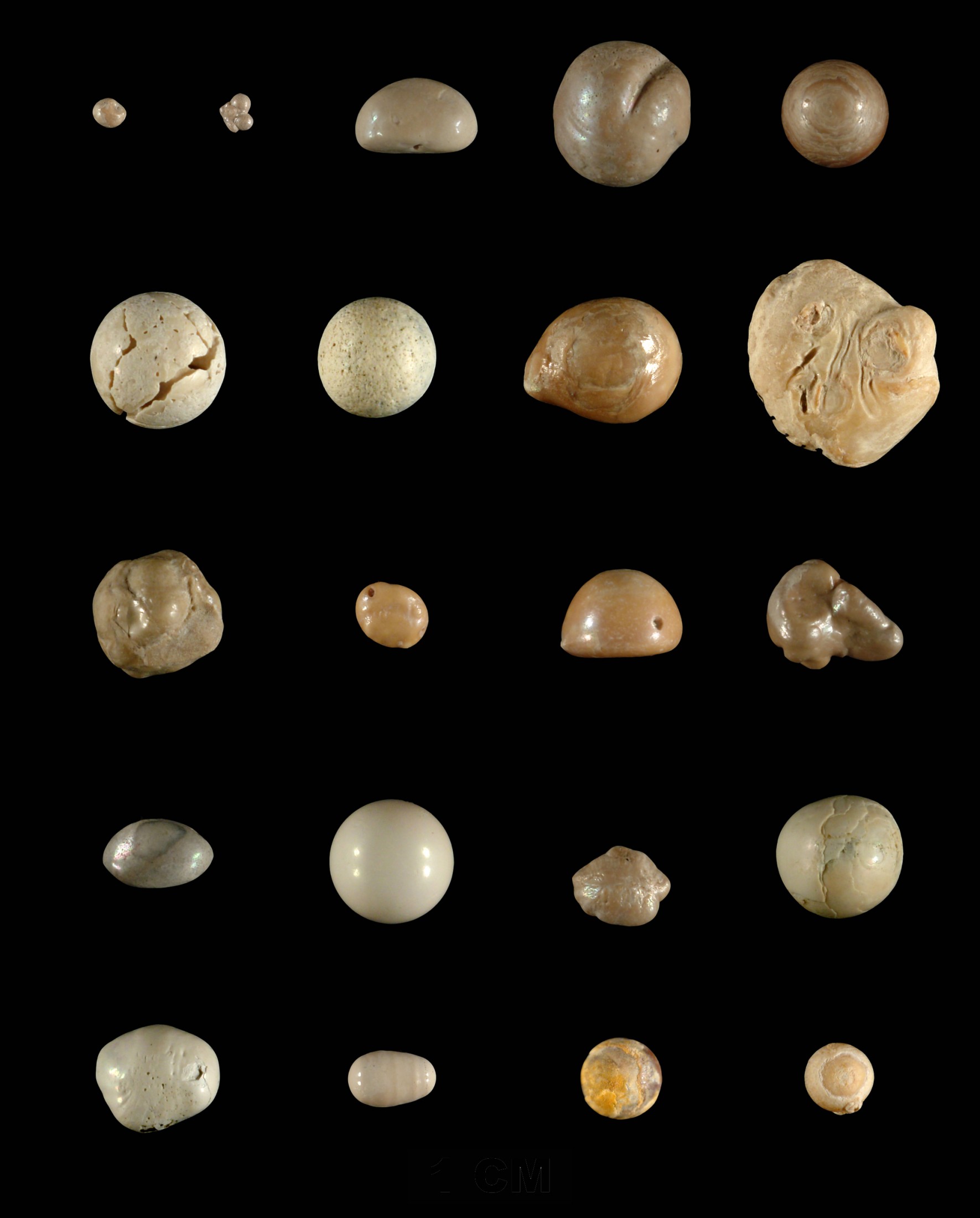The image depicts a meticulously arranged rock collection on a completely black background, possibly black cloth or black painted table. There are a total of 21 rocks organized in a grid pattern: the top row has 5 rocks, and the subsequent four rows each have 4 rocks, all spaced evenly apart. The rocks vary widely in terms of shape, size, color, and condition – some are perfectly intact, while others are damaged or fractured. The color spectrum ranges from white to tan to brown, and the rocks exhibit an array of textures and forms, from circular to oval and uniquely irregular shapes. This detailed and orderly arrangement suggests it could belong to a rock collector or scientist, possibly for research purposes.